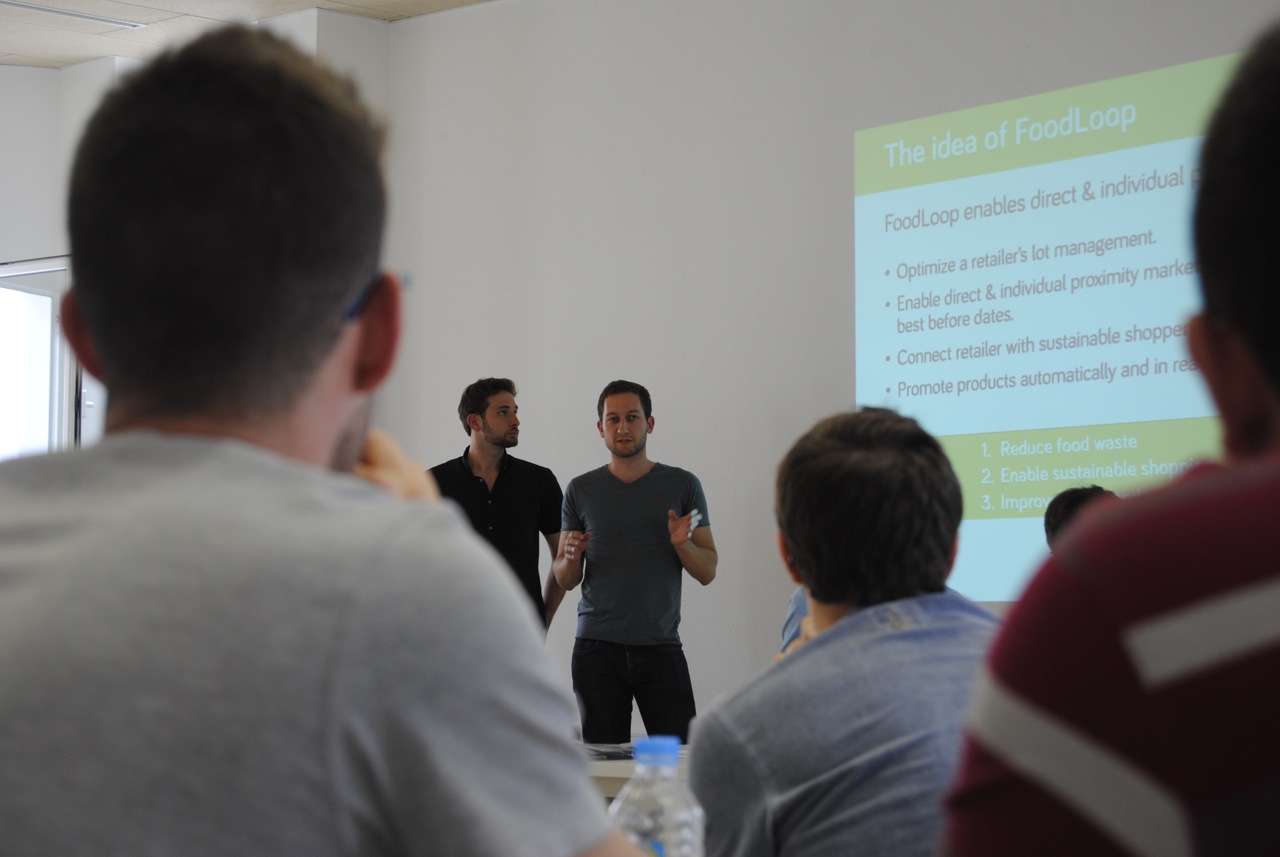The image depicts a business presentation being delivered by two men, both white and approximately 30 to 40 years old. The man on the left has short black hair, beard stubble, and wears a black button-down shirt with his hands on his hips. The man on the right also has short black hair, beard stubble, and is dressed in a grey t-shirt and jeans. They are presenting in front of a projected screen on a white wall, which has the title "The Idea of Food Loop" accompanied by bullet points discussing the benefits of the concept, including optimizing retailer lot management, enabling direct and individual proximity markets, highlighting best before dates, connecting retailers with sustainable shoppers, and promoting products automatically. The slide’s design includes a green banner and white background. An audience of at least four people, some with visible water bottles, is attentively watching. The text at the bottom of the slide highlights the goals of reducing food waste and enabling sustainable shopping, although parts of the text are obscured by the audience.